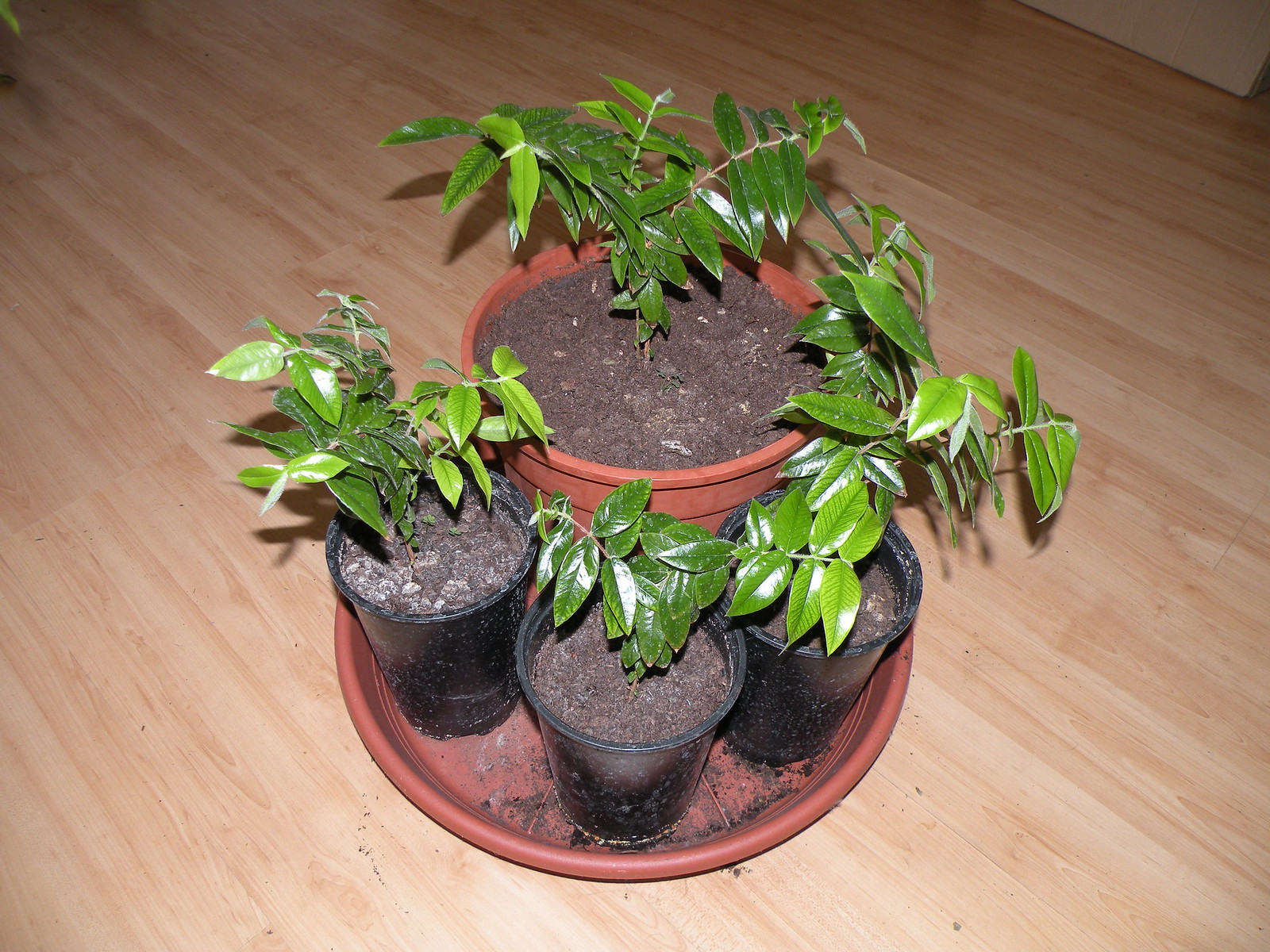The photograph features four small plants arranged in a terracotta-colored planter tray. Three of the plants are situated in smaller black plastic pots, while the fourth, slightly larger plant occupies a traditional terracotta pot. The plants exhibit a variety of green hues, including shiny light green and dark green leaves, some appearing waxy. The soil mixture in the pots includes dirt, gravel, and possibly some sand. A bit of soil has spilled into the planter tray and onto the light brown hardwood floor beneath it. The hardwood floor suggests an indoor setting. The flash used in the photo highlights the glossy texture of the leaves, adding a vivid contrast. In the background, the bottom corner of a wall is faintly visible, further hinting at an indoor environment.